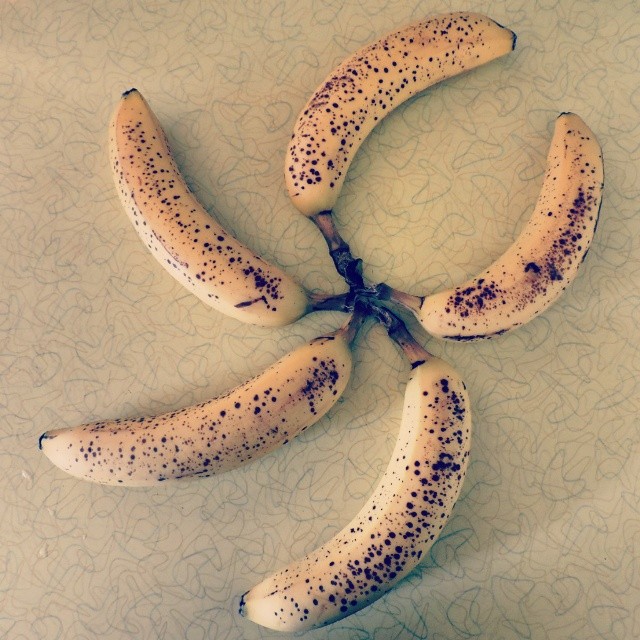In this photo, there is a tan-colored surface scattered with blue and purple squiggly lines, resembling random pencil scribbles. Five very ripe, yellow bananas with prominent brown speckles form a star-shaped pattern on this background. The bananas are particularly ripe, indicated by their numerous brown spots and blackened stems, a few days past their prime ripeness. The banana positioned at the bottom and the one towards the right show more speckling than the others. The background has a crackly texture with subtle blue or black lines running through the yellow, adding an artistic touch to the composition. There are no additional details, texts, or timestamps in the image.